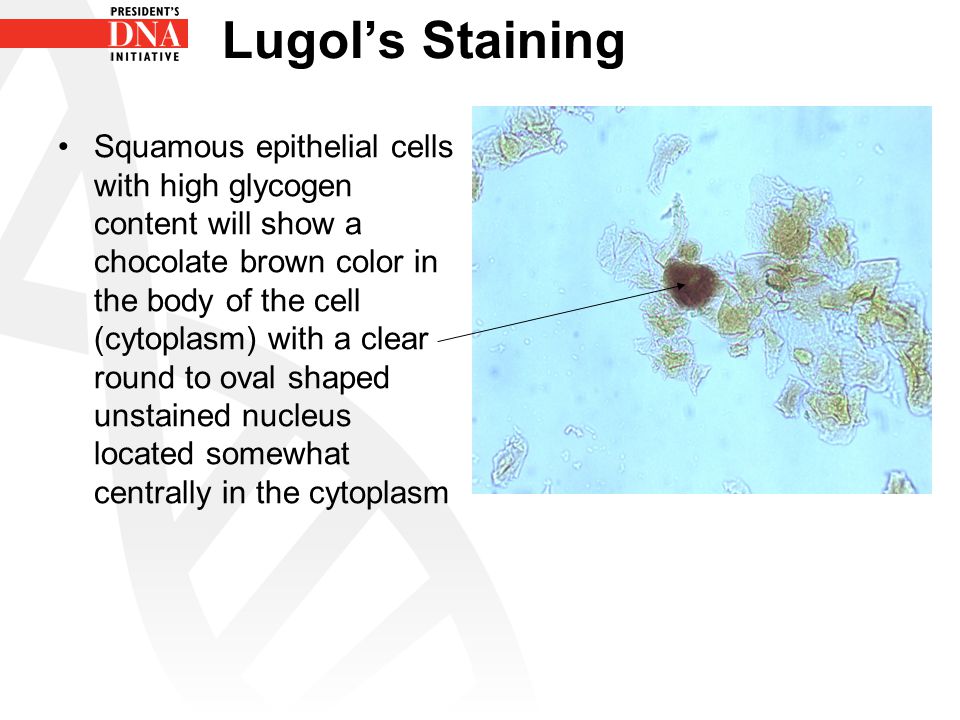**Lugose Staining:**

The image, titled "Lugose Staining," is a detailed medical photograph showcasing squamous epithelial cells with high glycogen content. A notable feature of these cells is that the glycogen-rich cytoplasm stains a chocolate brown color, while a clear, round to oval-shaped unstained nucleus is positioned somewhat centrally within each cell. The picture is set against a light blue background with some darker blue stains and contains cell structures with a prominent brown patch centrally located, surrounded by green and light brown fragments.

In the top left of the image is a small label stating "president's DNA initiative" inside a long red rectangle with white letters "DNA" and black letters underneath. To the right of this label and in black lettering, it reads "Lugol's staining," followed by the description of the squamous epithelial cells indicating their characteristic chocolate brown cytoplasm and centrally located unstained nucleus. The photograph provides a vivid representation of these cellular features as seen under a microscope, emphasizing the specific staining patterns used to identify high glycogen content in squamous epithelial cells.